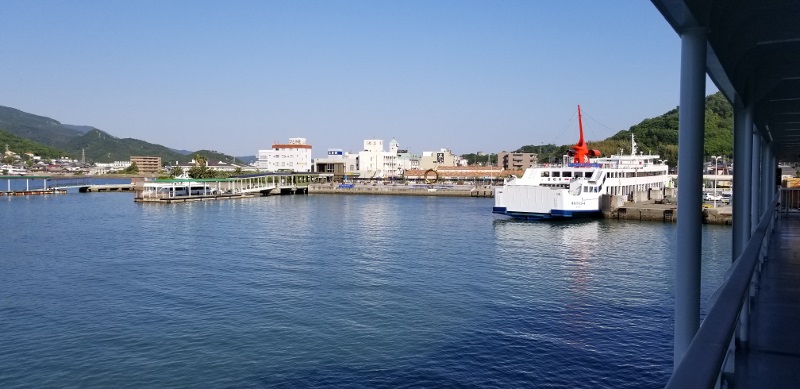In this vibrant outdoor scene, the image captures a serene lakeside view under a clear, blue sky. Dominating the foreground, a large white ferry boat adorned with numerous windows is docked beside a long gray deck, with a red structure visible on its top. Surrounding this central vessel are several smaller boats, contributing to the bustling maritime atmosphere. A bridge with white pillars spans the water from where the photo is taken, adding structural elegance to the scene. The backdrop features a lush, green hill dotted with trees, while a distant mountain range softly frames the horizon. In addition to the natural beauty, the shoreline is lined with a mix of buildings, encompassing white condos or apartments and some brick structures—possibly hospitals or other significant establishments. Despite the charming water setting, an array of unarranged elements, including possibly scattered debris, add a cluttered aspect to this quaint beach town.